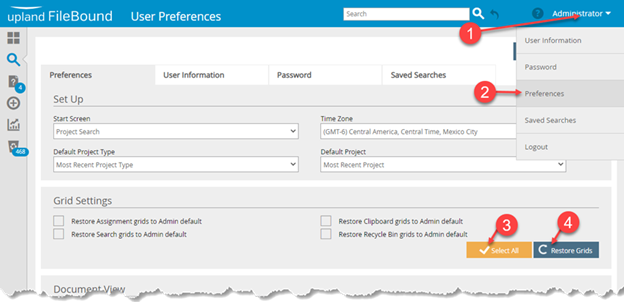The image is a screenshot of a user preferences configuration page within the Upland FileBound system, characterized by a variety of interface elements and annotations. 

At the very top, there is a prominent blue banner displaying the title "Upland FileBound User Preferences." Just below this banner sits a search bar for navigation. On the top-right corner, there's a section labeled "Administrator," highlighted by an annotation with the number 1 and a red arrow pointing to it.

The main portion of the screen is divided into several sections. The selected tab is "Preferences," under which the user can configure "User Information," "Password," and "Saved Searches." An additional drop-down arrow under the "Administrator" section reveals options for "User Information," "Password," "Preferences," "Saved Searches," and "Logout." 

The central area of the screen titled "Setup" lists various configurable settings including "Start Screen," "Project Search," "Time Zone" (specified as GMT-6, Central America, Central Time, Mexico City), "Default Project Type," "Most Recent Project Type," "Default Project," and "Most Recent Project." Additional options include "Grid Settings" with actions like "Restore Assignment Grids to Admin Default," "Restore Search Grids to Admin Default," "Restore Clipboard Grids to Admin Default," and "Restore Recycle Bin Grids to Admin Default."

At the very bottom right, two prominent action buttons are visible. The first is an orange rectangle labeled "Select All" in white text, annotated with a number 3 and a red arrow. Next to it is a blue rectangle labeled "Restore Grids" in white text, marked by an annotation numbered 4 with a red arrow pointing towards it. The bottom edge of the screenshot features a deliberately torn visual effect, adding a unique design element to the image.